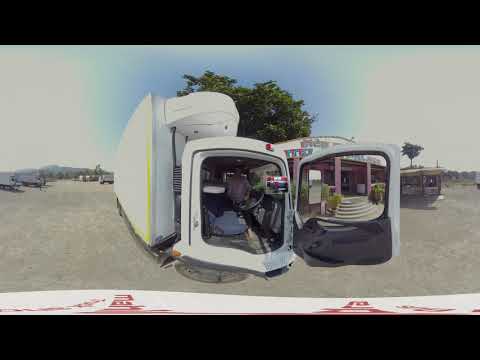The image captures an open door on the cab of a large vehicle, possibly a truck or a food truck, with the frame of the door painted white. Inside the door, there's a black strip of insulation and a dark floor with light illuminating the foot area. A black bag hangs from the bottom of the door, while a gray bag rests on the floor. Through the window of the open door, a building with purple poles holding up a roof and rounded stairs leading to the entrance is visible. The background above the building and tree transitions from blue to white. The ground around the vehicle appears to be a light gray or gray dirt area. A person is discernible inside the cab near the steering wheel. Additionally, the image has black borders on the top and bottom, and illegible red and white writing at the bottom. There are a couple of trailers parked in the background to the left and another building with a tree on the right.